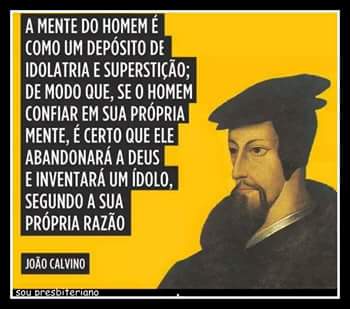This image appears to be a digital meme or artwork with a white border against a thicker black border. The main focus is a classical-style painting of John Calvin, identifiable by his distinct features: thin eyebrows, almond-shaped eyes, a long, combed goatee beard, and a black beret atop his head. He wears a black jacket over a white collar and has fair skin with a long nose, staring expressionlessly. This artistic rendition against a completely yellow background includes various overlays of white text within black rectangles. To the left of John Calvin, the largest text, possibly in Spanish, stands prominently, followed by smaller text that reads "João Calvino," a Portuguese version of John Calvin. Below this, another black rectangle contains text stating "Sous Presbyterian," likely translating the term 'Presbyterian.'